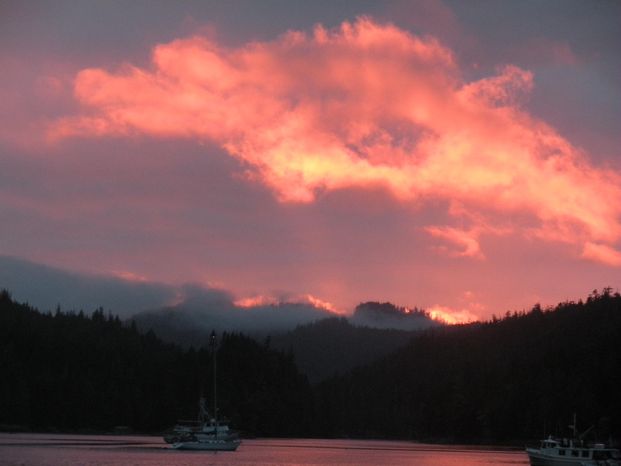This horizontal photograph captures a breathtaking sunset over a serene body of water, possibly a lake or river, framed by a wooded shoreline and nestled mountains in the distance. The sky dominates the image with a dramatic explosion of colors, featuring deep gray clouds interspersed with vibrant hues of orange, yellow, and pink, creating the illusion that the sky is on fire. The vivid tones of the sunset are reflected in the calm water below, adding to the scene's mystique and tranquility. Two boats, one in the lower right and another in the lower left, gently sail on the water, contributing to the peacefulness of the moment. The mountains in the background are partially shrouded in mist, enhancing the depth and beauty of the landscape. The sun has dipped below the hills, casting a soft glow and signaling the approach of night, making for a stunning and serene visual experience.